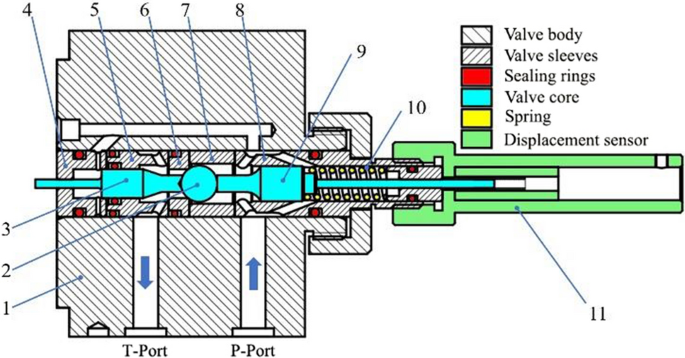This is a computer-generated diagram depicting a cutaway view of an unidentified mechanical device, likely a valve. The drawing features a simple line schematic characterized by numbered labels from 1 to 11 pointing to various components. Each part is distinctly highlighted with different colors or patterns to correspond with a legend situated in the upper right-hand corner. The legend identifies key components such as the valve body, valve sleeves, sealing rings, valve core, spring, and displacement sensor. The diagram shows a square central body with various pieces protruding from and entering it, including a distinct green-colored part.